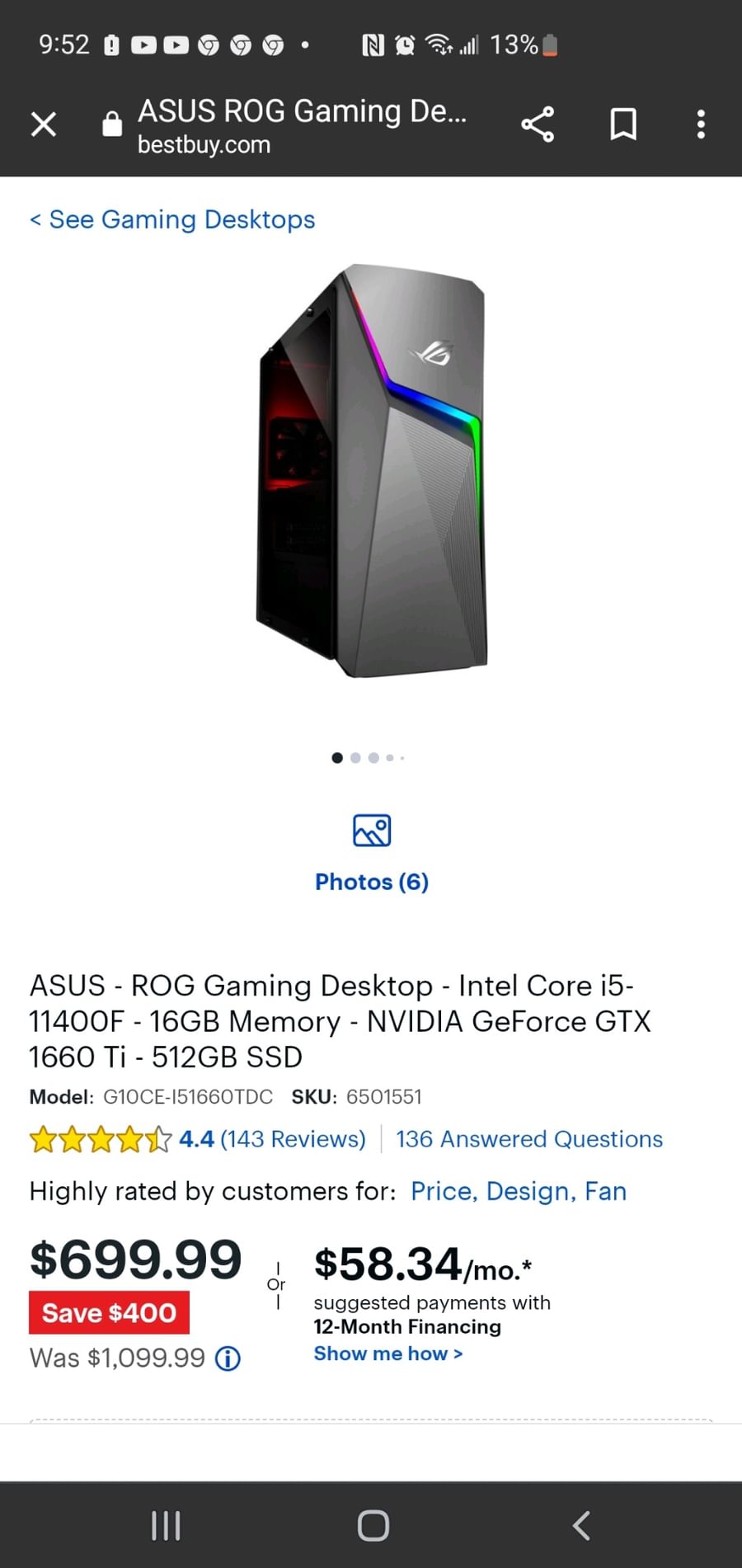A person is browsing BestBuy.com on their smartphone and looking at an ASUS ROG Gaming Desktop. The specifications of the computer are highlighted, showcasing an Intel Core i5-11400F processor, 16 GB of memory, and an NVIDIA GeForce GTX 1660 Ti graphics card. It also features a 512 GB SSD for storage. The product has a rating of 4.4 stars, based on 143 reviews, and 136 customers have answered questions about it. It is highly rated by customers for its price, design, and cooling fan. The regular price of the desktop is $1,099.99, but it is currently on sale for $699.99, providing a savings of $400. Additionally, there’s an option for 12-month financing with suggested payments of $58.34 per month.